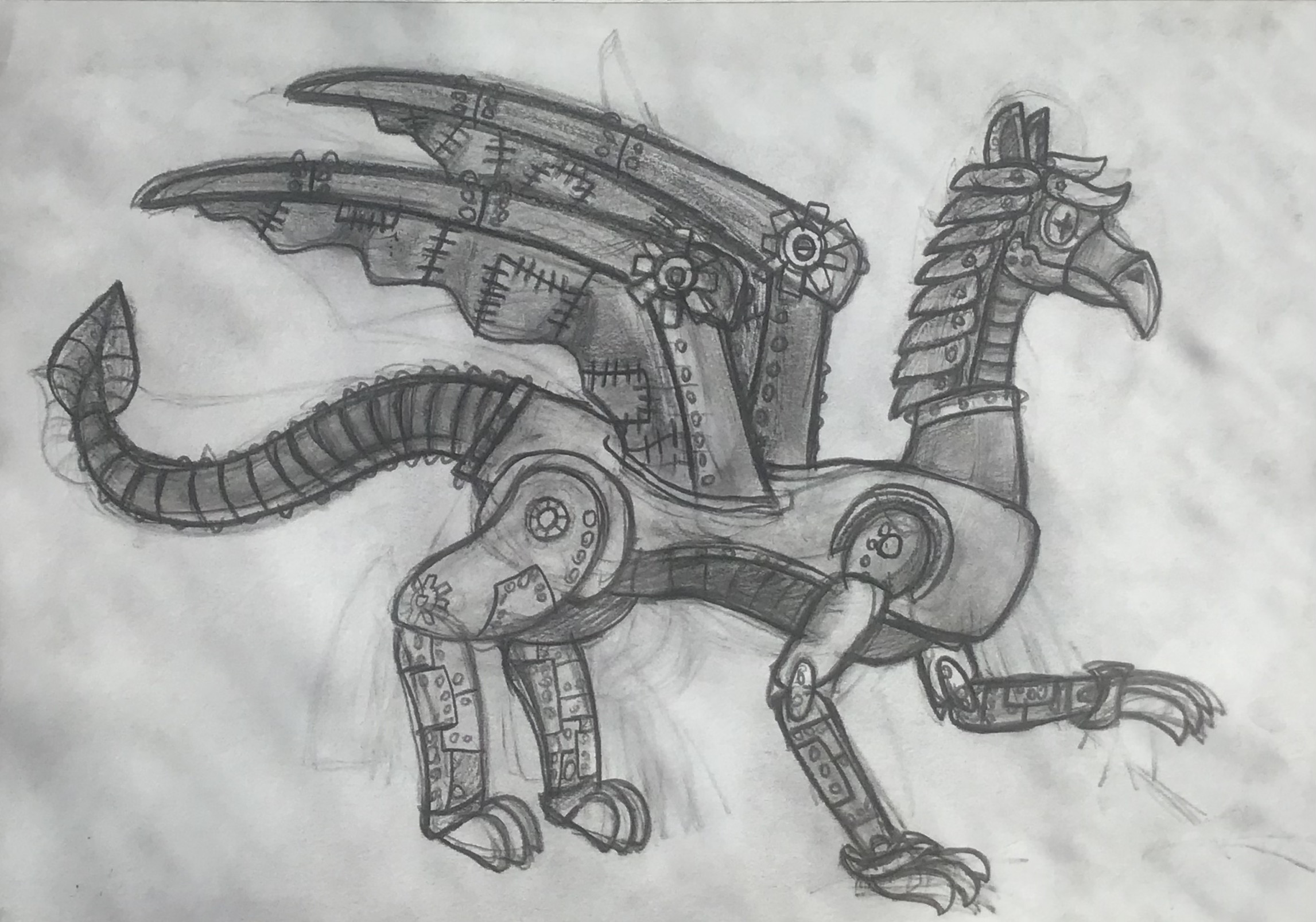This detailed pencil sketch features an imaginative, steampunk-esque creature that merges elements of a dragon, lizard, bird, and robot. Set against a lightly clouded, misty background created with delicate pencil streaks on white paper, the figure stands out in graphite gray. The creature has four mechanical feet, each ending in talon-like claws. Its left front leg is raised and bent at a 90-degree angle, with elbows pointing backward, while the other three feet remain grounded. The tail is segmented and ends in a rounded, pointy leaf-like shape. Two wavy wings, bent at a 70-degree angle, extend from its body, which is joined together with what appear to be rivets or gears. The head resembles a horse or dragon, featuring a pointy beak, a plume of fur or feathers along its tall neck, and two pointy ears atop its head. The creature looks to the right with its tail pointing left, giving the impression of mid-step motion, suggesting a whimsical but mechanical bird-like figure. The overall drawing, though not a masterpiece, showcases the competent skills of a possibly young artist, evoking a sense of a high school student's inventive classroom doodle.